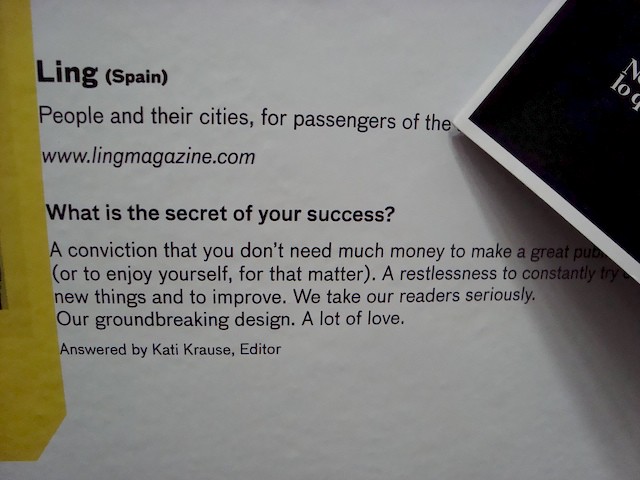The image depicts a piece of paper featuring text in black on a white background. At the top, in bold black letters, it says "Ling" with "(Spain)" in parentheses next to it. This is followed by partially obscured text that begins with "people and their cities for passengers of the," with the latter part blocked by an overlapping black card with a white border, casting a shadow on the page. There is a web address in italicized font, "www.lingmagazine.com," and beneath that, in bolder print, a posed question: "What is the secret of your success?" The response reads, "A conviction that you don't need much money to make a great," and the rest of the sentence is cut off. It continues, "or to enjoy yourself, for that matter. A restlessness to constantly," before being cut off again, likely continuing with "try new things and improve." The final legible sentences state, "We take our readers seriously. Our groundbreaking design. A lot of love." It is noted at the bottom that the answer was provided by "Katie Krause, editor." The left side of the image features an overlay of a gold-colored sheet, adding a layered dimension to the photo, which appears to be a photograph rather than a scan.